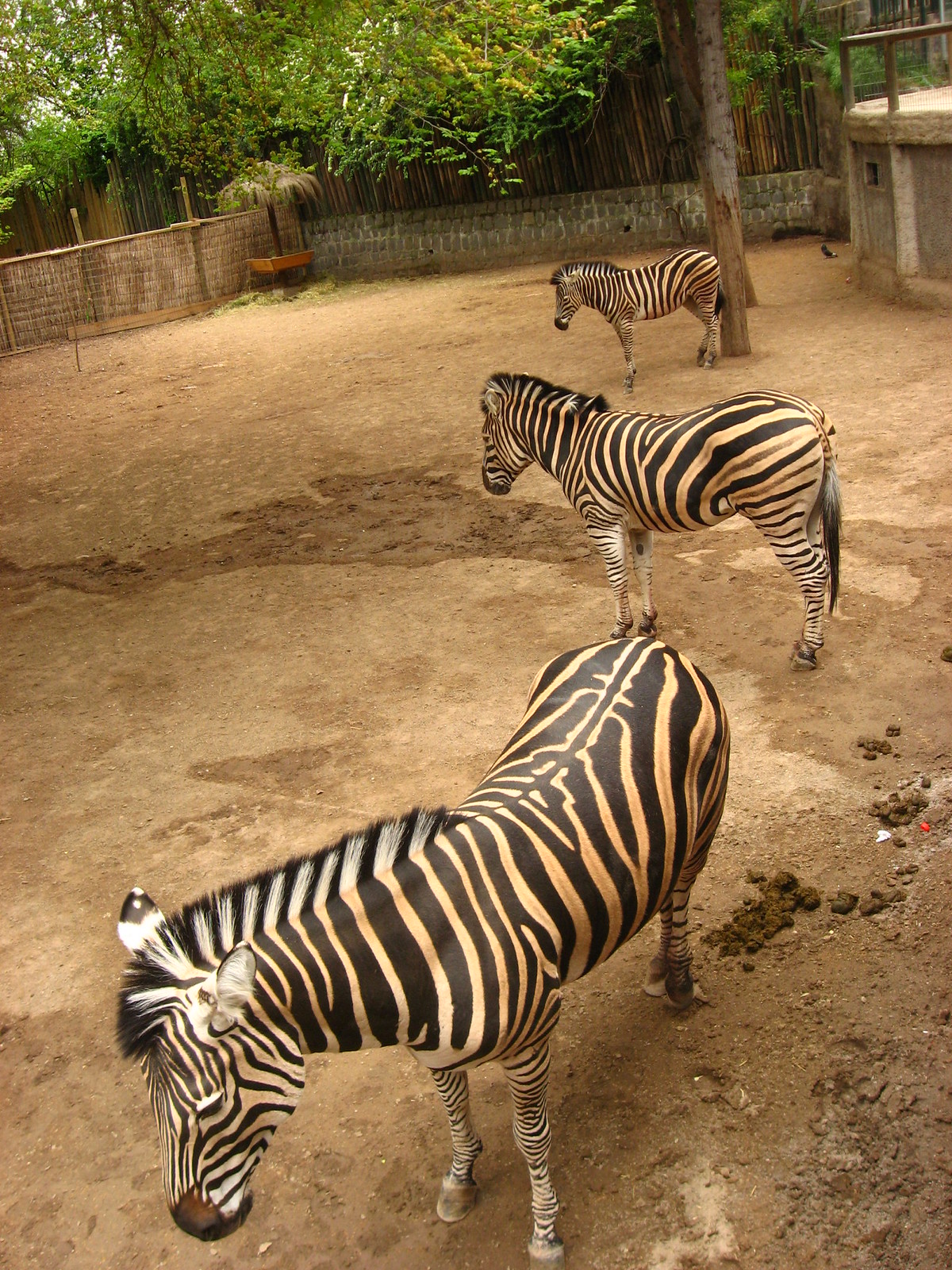The photograph showcases three zebras standing on a dusty, light brown dirt ground in a zoo enclosure. The enclosure features a cobblestone brick wall and a woven, reed-style fence on the left, with a tall wooden fence running along the back. Overhanging foliage and trees are visible beyond the fencing, adding a touch of greenery to the scene. A small manger filled with hay is tucked in the back corner. The zebras, all adorned with their distinctive black and white stripes, are positioned in a line: one in the foreground, one in the middle, and one toward the back, near the lone tree in the enclosure. The two zebras in the back face left, with their heads slightly bowed, while the zebra in the front center looks more toward the camera, offering a calm and serene presence. Patches of wet ground and some droppings are also visible, adding to the natural and uncensored environment of the scene.